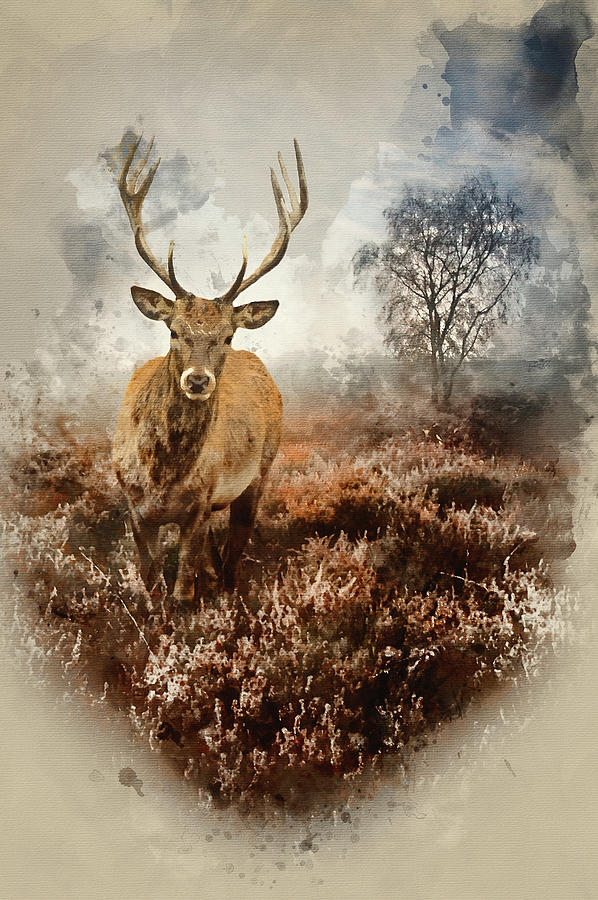The image presents an exceptionally detailed and realistic depiction of a male deer, or buck, set within an intricate landscape. The deer, with its prominent brown antlers and deep, gazing eyes, looks directly at the viewer, exuding a serious demeanor. Its fur, richly textured and lifelike, showcases a mix of brown tones with lighter patches on the belly and white accents around the black nose. The alert ears stick out just below the majestic antlers. The buck stands amidst a mix of dried brown and white grass, dotted with some flowering plants.

In the backdrop, a blend of a brownish landscape and grayish off-white hues prevails, adding to the picture's somber tone. Blue-gray clouds mix with mist and fade into the gray background, creating a washed-out effect. A distant tree with gray leaves can be seen through the mist. The setting further includes what appears to be water below the deer, accentuated by a few floating leaves, with the overall coloration dominated by earthy tones of black, white, gray, brown, and blue. The composition is meticulous, with each element contributing to the lifelike and serious character of the scene. No other animals or people are present, and the scene is devoid of any text.